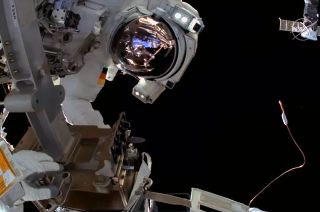In this low-resolution image, the central focus is on an astronaut positioned in the upper left corner. The astronaut appears slightly upside down and on their side, with their reflective helmet visor on, casting a gleam amidst the surrounding darkness. The background of the image is pure black, devoid of any stars or celestial objects. The astronaut is intently looking down into a complex array of machinery, which includes a gray bar with a cylindrical attachment and some brown metal components. Another astronaut is partially visible, identifiable by their gloved hand touching one of the brown parts, suggesting they are assisting with the task. This assisting astronaut's glove points up from the lower portion of the image. Additionally, there is a small antenna or wire emerging on the right side and a tiny satellite visible in the top right corner, indicating the presence of other equipment in this space environment.